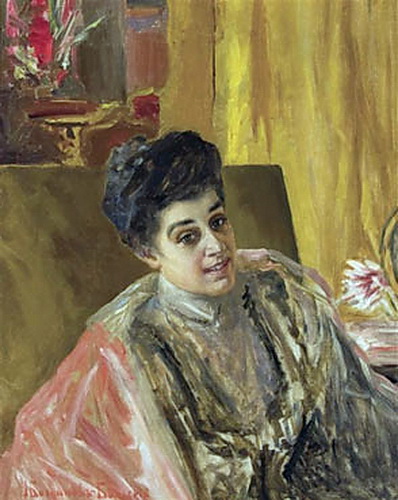This vertically aligned rectangular painting features a Renaissance-style depiction of a woman with her dark hair styled in an elegant updo, possibly a bun, adorned with a headpiece at the back. Her expressive face, with slightly raised black eyebrows and brown eyeshadow, is turned towards the left as she smiles, revealing her teeth. She is draped in an ornate attire: a gold and white garment, complemented by a flowing pink and white cape. The woman appears to be seated on a cushioned, rectangular brown chair, reminiscent of antique furniture from older eras, possibly the 1500s. The background is a mixed display of a yellow and brown-streaked wall, adding a touch of aged texture. On the right side of her, on a table adjacent to the chair, rests a pink and white flower, meticulously drawn. In the upper left corner of the painting, there is an abstract representation of a vase with additional pink and white flowers, portrayed with a color-block style that emphasizes different shades of wood grains.